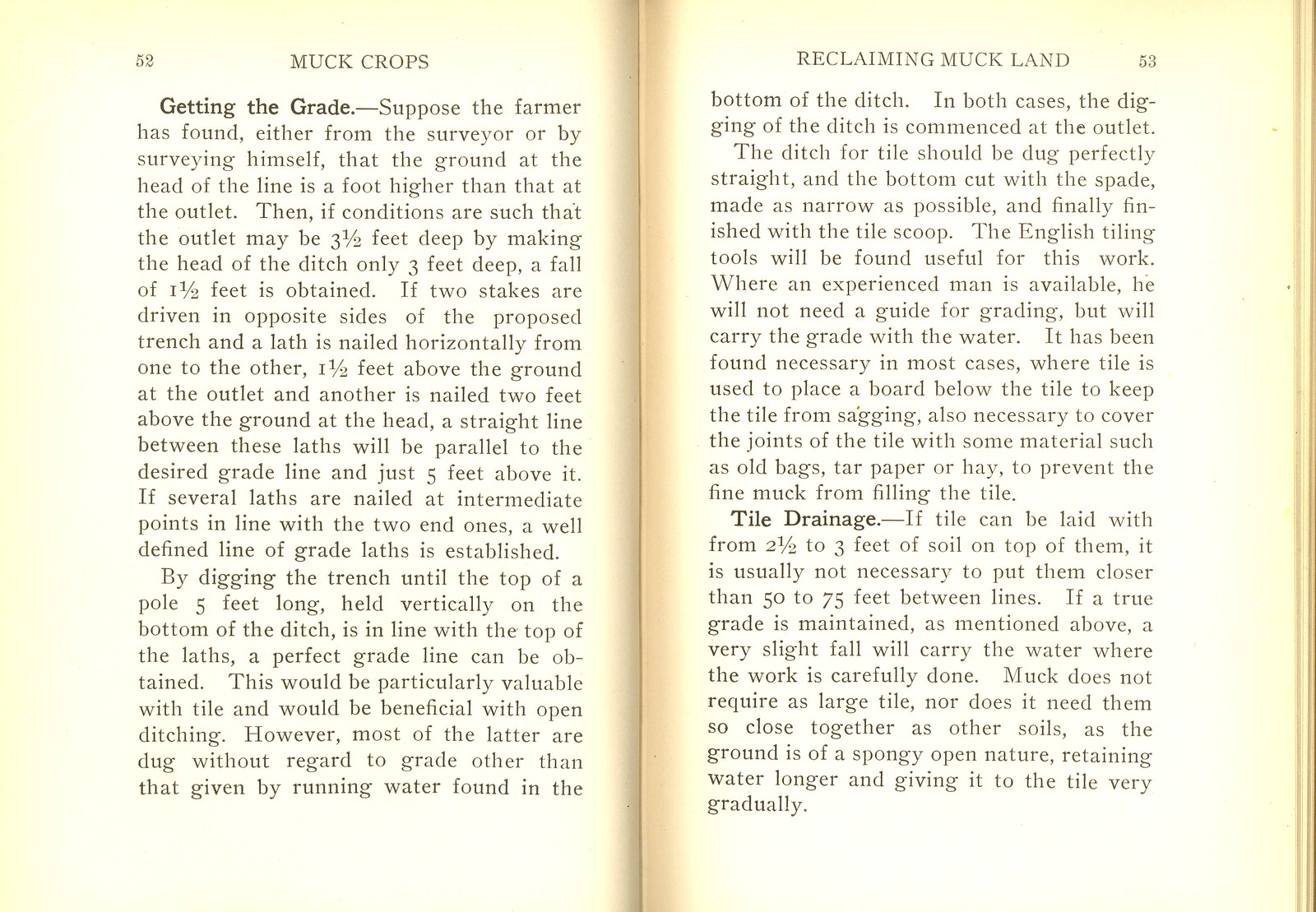This photograph captures an open book displaying pages 32 and 33. The pages are noticeably withered and yellowed with age. The left page features the header "Muck Crops," while the right page is titled "Reclaiming Muck Land." The detailed text spans various farming techniques, specifically addressing the processes and conditions essential for cultivating muck crops and reclaiming muck land. It provides instructions on the necessary trench digging, detailing the required trench depths for beneficial ditching, and continues with guidelines on tile drainage, specifying optimal distances between 50 to 75 feet.